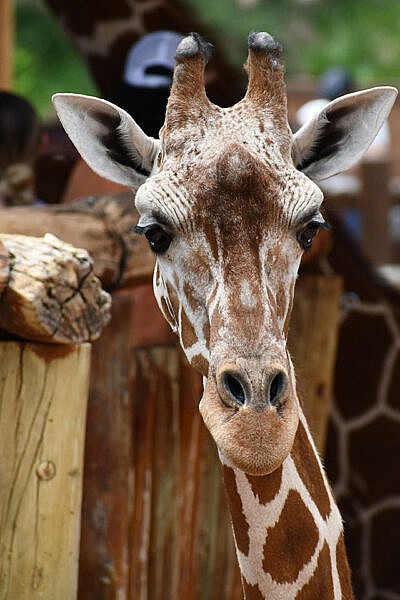This is an up-close photograph of a giraffe's head and a portion of its neck. The giraffe's coat features its characteristic brown patches set against a cream-colored background. Its large, round eyes are a deep brown, with its pointy ears—white on the outside and black on the inside—perked attentively. At the top of its head are the giraffe's ossicones, which are brown at the tips and have black markings. The giraffe has a small bump between its eyes and flared nostrils, and it appears to be looking directly at the camera. The background is blurry, revealing a wooden structure and hints of greenery. Also behind the main giraffe, a second giraffe can be partially seen, along with a person wearing a baseball cap.